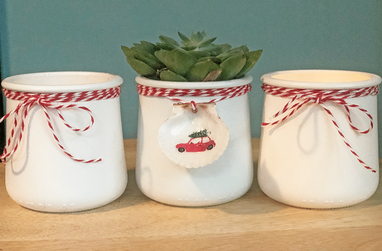This horizontally-aligned rectangular image features three identical, wide-mouthed white containers, resembling coffee mugs but without handles, displayed on a light brown wooden surface. Set against a dark green wall, these containers are adorned with red and white candy cane-patterned ribbons tied around their tops. The container on the left and the one on the right are both empty and have their ribbons tied in neat bows at the front. The central container stands out with a lush, densely-packed plant featuring short, vibrant green leaves protruding from its wide mouth. Additionally, a circular ornament affixed to its ribbon showcases a charming design of a red car with a Christmas tree on its roof, adding a festive touch to the scene, giving an impression that they might belong in a kitchen or a holiday-themed setting.